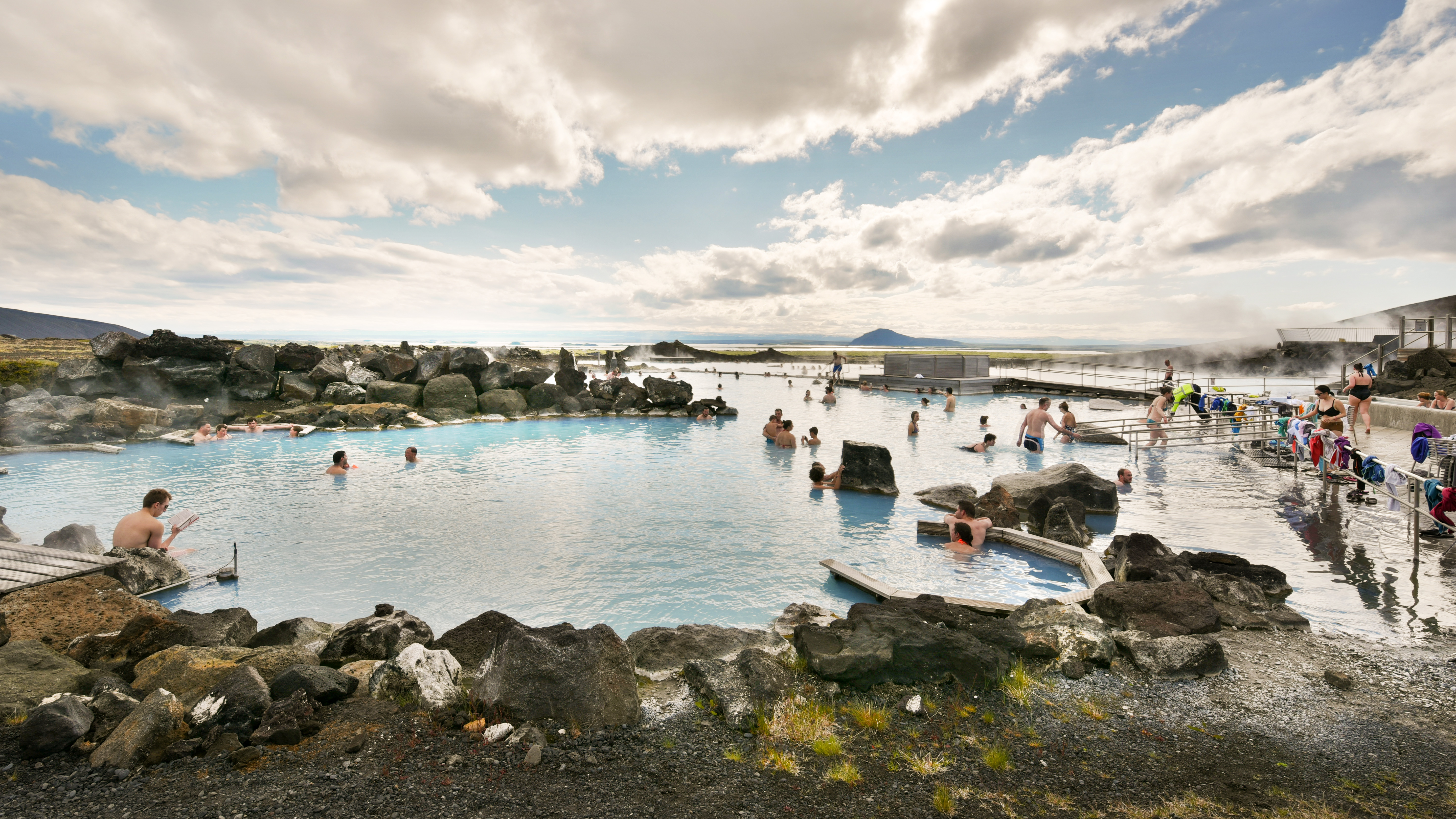In this vivid image, several people enjoy a bright, sunny day at what appears to be a pristine hot springs or natural lagoon, possibly the Blue Lagoon. The blue, shallow water is surrounded by black and gray rocks, some covered with moss, creating a striking contrast with the clear, sunny sky dotted with a few clouds. On the left side of the image, a wooden dock or walkway leads towards the water, while on the right, another walkway extends into the lagoon, perhaps connected to a small bathhouse. Steam rises from the water, adding to the serene atmosphere. Both adults and children can be seen enjoying the water, with clothing and personal belongings hanging on a rail nearby. The abundance of people and the well-built walkways hint at the location being a popular and well-maintained spot for relaxation and recreation.